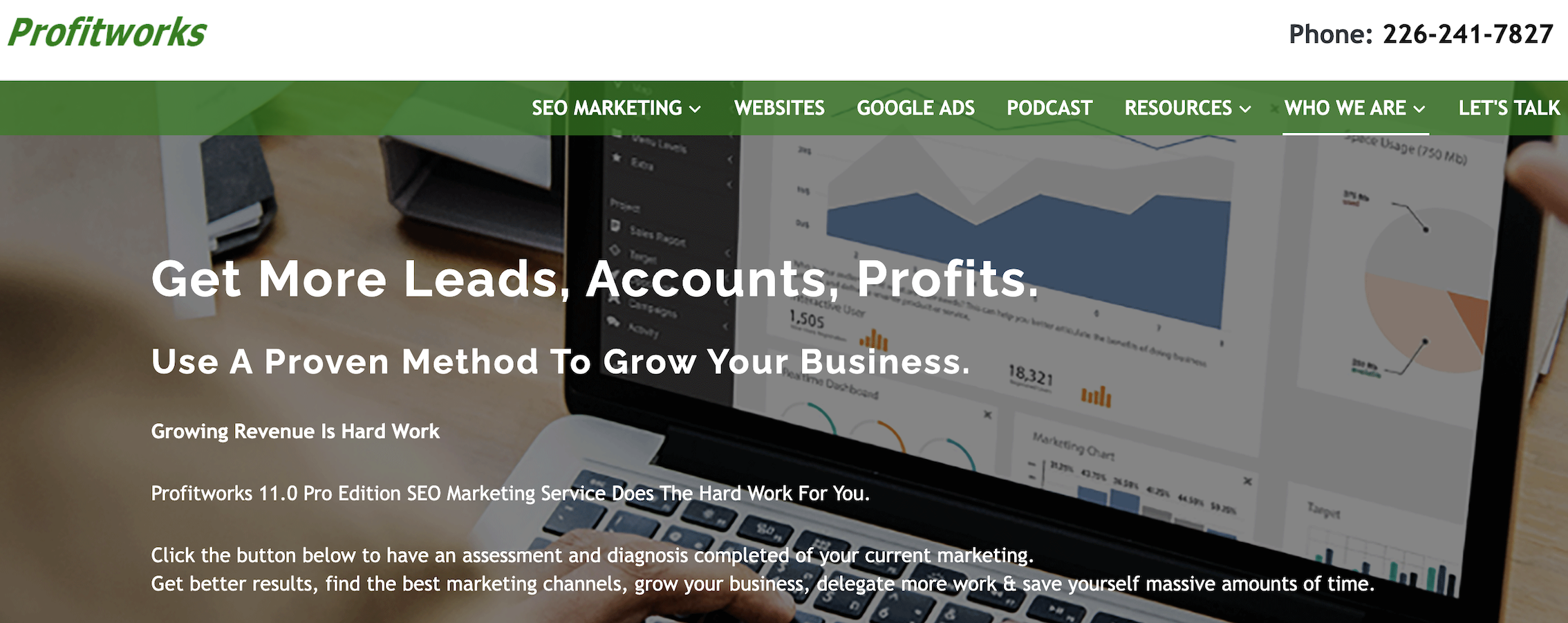Here is a detailed and cleaned-up descriptive caption for the image:

---

The image, sourced from the ProfitWorks website, features a prominent green banner at the top displaying navigation options such as SEO Marketing, Websites, Google Ads, Podcasts, Resources, Who We Are, and Let's Talk. Below this banner, there is a high-resolution photograph of an open laptop. The laptop screen displays various charts, graphs, and financial data, with an individual's hand actively working on it. Superimposed over the laptop image is white text that reads: "Get more leads and accounts, profits, use a proven method to grow your business."

Beneath this visual, a brief description elaborates on the company's offerings related to marketing and business growth. The image suggests a call-to-action, prompting viewers to click a button for an assessment and diagnosis, although this button is not visible in the snapshot. In the top right corner of the image, the company's phone number is prominently displayed, reinforcing the call-to-action element. This visual serves as a strategic sales pitch from ProfitWorks, aiming to attract potential clients with the promise of increased leads and business development.

---